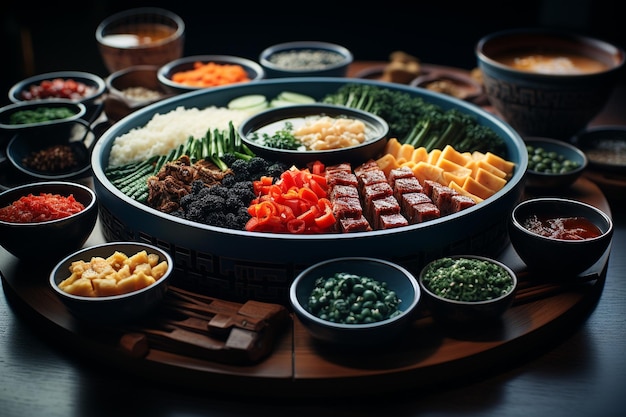The image depicts a vibrant charcuterie spread arranged on a large circular dish that functions similarly to a Lazy Susan, with a dark wooden base that can be spun. The dish is filled with a diverse assortment of foods including meat cubes, cheese, brightly colored vegetables such as peppers, green beans, peas, and possibly even raisins and beets. At the center of the dish, there's a bowl containing a dip garnished with cheese and green onions. Surrounding the central circle are numerous smaller dishes – perhaps 14 or more – each containing a variety of other food items in vibrant colors ranging from reds and yellows to greens and whites. Notably, off to the side, there is a larger black bowl that could be holding soup or another type of dish. The overall presentation is colorful and eclectic, with all items clearly visible and well-lit, creating a visually appealing and appetizing scene.